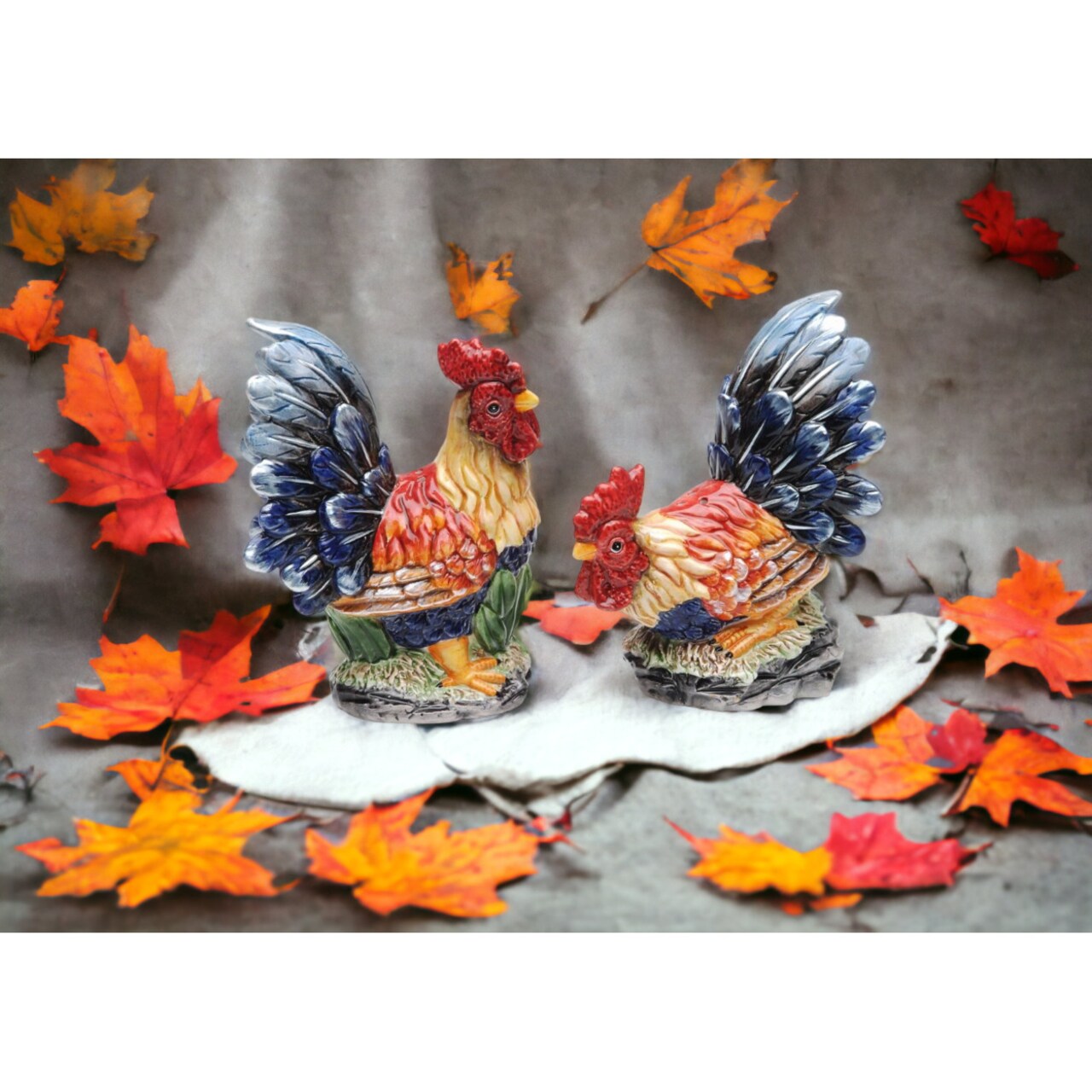The image captures two colorful ceramic roosters placed on a light, possibly white surface with a gray mat background. The roosters are surrounded by an array of vibrant fall leaves in shades of yellow, orange, and red, some of which appear blurred due to depth of field effects. The rooster on the left stands upright, featuring a red face, a red body, and a blue tail, while the rooster on the right, similarly colored with red, white, orange, blue, black, and yellow feathers, is leaning forward with its face down. Both roosters face each other, giving the scene an intimate and festive atmosphere reminiscent of autumn and Thanksgiving decorations.